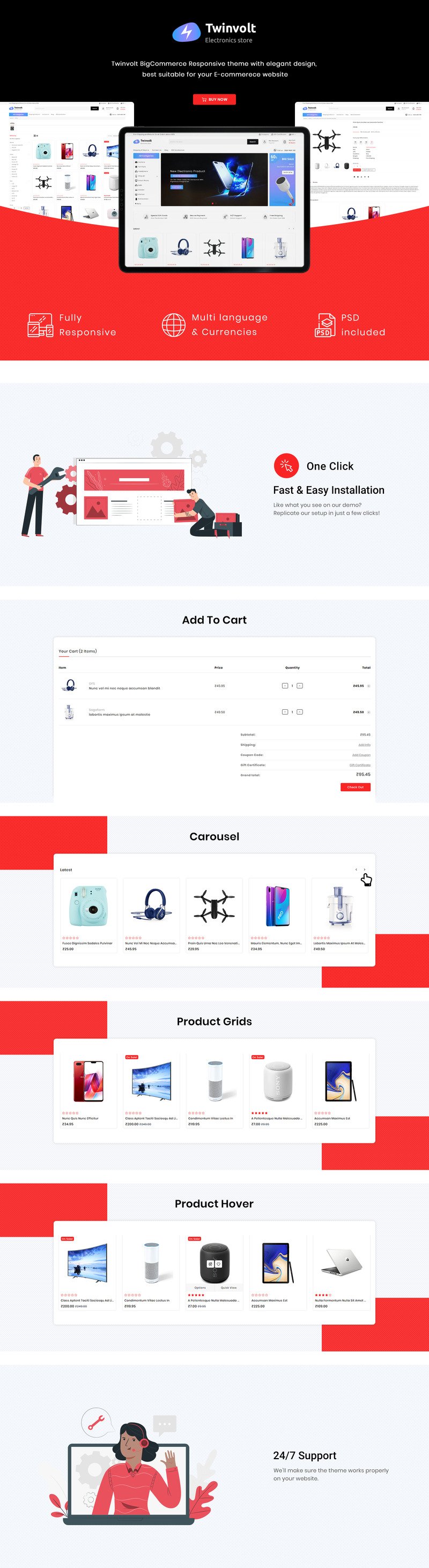Here's a cleaned-up and detailed caption for the image:

---

The website showcases a variety of products for sale under the brand name "Twinvolt," prominently displayed in white at the top of the page. It is identified as an electronic store specializing in e-commerce solutions, featuring the tagline "Twinvolt: Big E-commerce Responsive Theme with Ellica Design, Best Suitable for E-commerce Websites." 

Below this, there is a red "Buy Now" button centrally located, accompanied by snapshots previewing various items available for sale, complete with descriptions and prices listed beneath each product. 

In the middle section, an iPad displays the website interface, and another image below features a drone with the caption "Fully Responsive" on a red background. This section highlights features such as "Multiple Languages and Currencies," represented by a globe icon, and notes that a PSD file is included.

Further down, an image depicts a man with a large wrench in front of a settings page, emphasizing "One-click Fast and Easy Installation." Adjacent to this, there is an "Add to Cart" box showing a preview of items in the cart, including options to adjust quantities, view the subtotal, and see a price breakdown.

Below this, a carousel displays a collection of miscellaneous items like Coolpix cameras, headphones, and drones. This variety is complemented by a product grid featuring five images. Each product in this grid is presented with a star rating, a detailed description, pricing information, and a note indicating "24/7 Support."

To the left of the product grid, an image of a woman wearing a headset with her hand raised underscores the availability of around-the-clock customer service support.